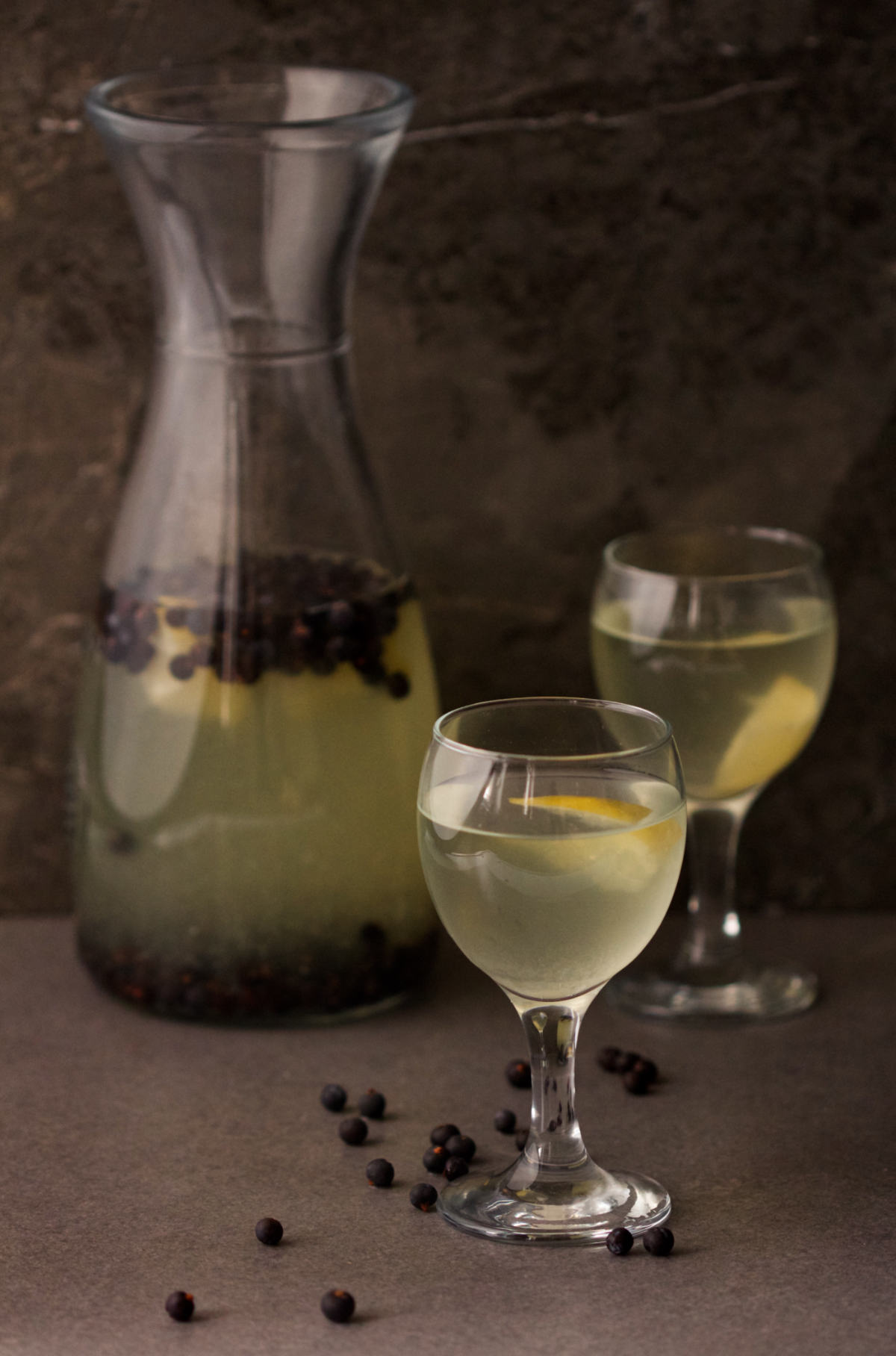The photograph features a large glass pitcher containing a cloudy yellow-greenish beverage resembling lemonade, with blueberries both floating on the surface and settled at the bottom. The pitcher is positioned on a light gray stone surface in front of a brown and black marbleized wall. Two wine-like glasses filled with the same yellow-greenish lemonade are situated to the right of the pitcher. The marbleized background and the gray stone table create a sophisticated setting, accentuating the contrast with the vibrant colors of the lemonade and blueberries, highlighting the intriguing mixture within the pitcher and glasses.